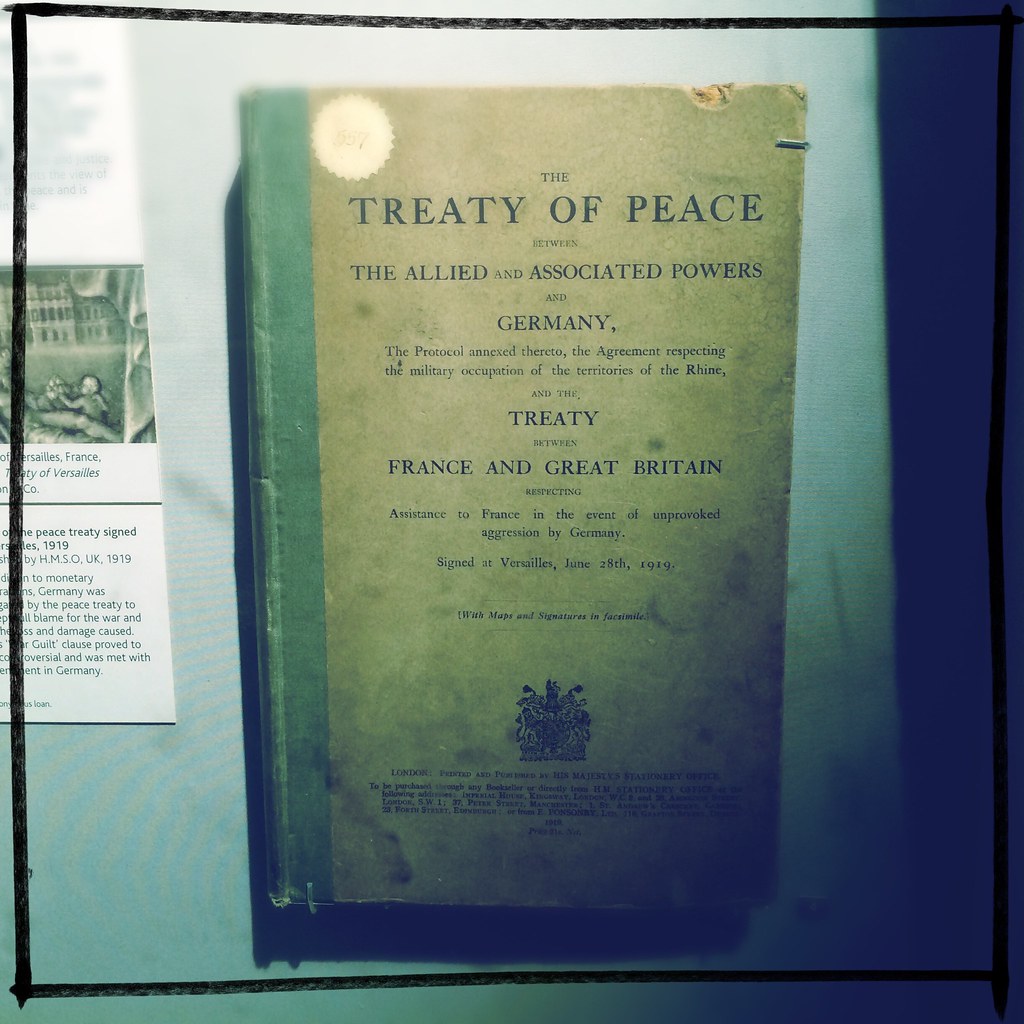This image features a very old, worn, hardcover book titled "The Treaty of Peace, the Allied and Associated Powers and Germany, the Protocol Annexed Thereto, the Agreement Respecting the Military Occupation of the Territories of the Rhine, and the Treaty between France and Great Britain, Respecting Assistance to France in the Event of an Unprovoked Aggression by Germany, signed at Versailles, June 28, 1919." The book, likely a first edition, shows significant wear with battered corners and a discolored cover, indicating its age. It has a green spine and features an emblem and the word "London" at the bottom, though parts of the text fade into darkness. The book is displayed behind glass, suggesting it is part of a museum exhibition. To the left of the book, there is an informational sign with an illustration, possibly of a historic city and a child, and text partially visible, mentioning "Peace Treaty Sign 1919, HMSO UK 1919" and "Germany." The background of the display is stark white, accentuating the age marks and imperfections of the book, which serve as a poignant reminder of its historical significance related to the end of World War I.